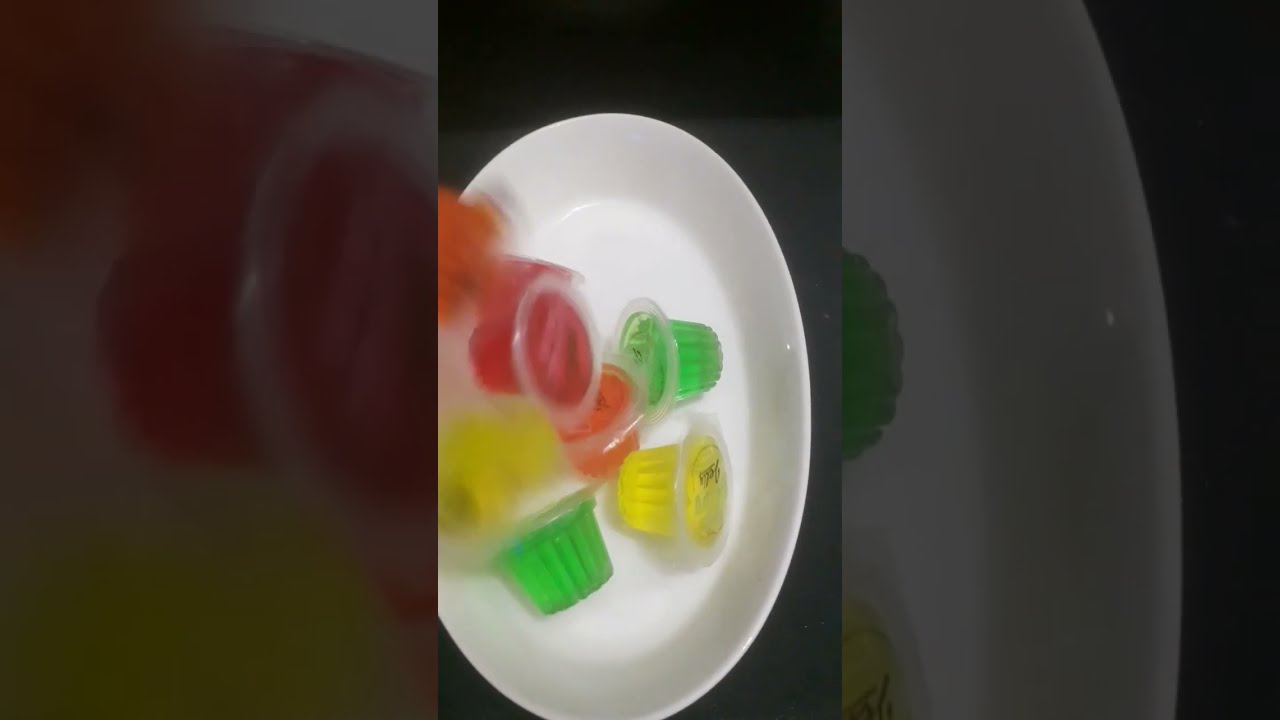The image depicts a collection of individually packaged jello cups arranged on a white, circular plate that is situated on a white table. The jello cups come in various vibrant colors: two green, two red, two orange, and two yellow, all sealed with a clear plastic cover. The photo is in portrait orientation and has a dark background, accentuating the plate in the center. This plate appears slightly taller than it is wide. Notably, the image includes an artistic effect wherein blurred versions of the jello cups seem to cascade onto the plate from the left, suggesting motion. The entire scene is overlaid with a translucent, zoomed-in version of the jello cups, tinted black, creating a layered visual effect. The combined imagery and color contrasts give the impression of a dynamic, possibly screen-captured moment, as if from a video or a social media post.